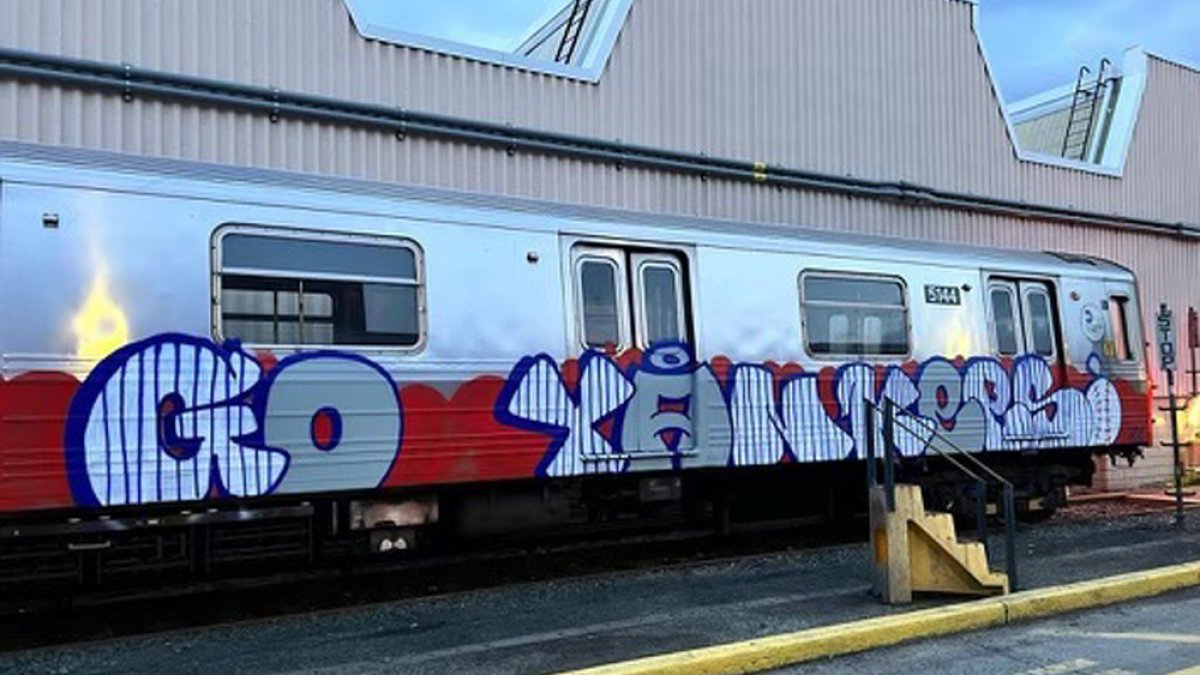The image depicts a silver subway train compartment situated near a warehouse-like building, identifiable by its distinct roof style. The train, facing left at a diagonal angle, features two doors, two rectangular windows, and the number "5144" clearly visible towards the far right. The lower part of the train is emblazoned with vibrant graffiti spelling out "G.O.A.N.K.E.S.S" in a dynamic, multi-colored style. The graffiti's letters display a pattern of blue, gray, and white hues with red outlines and solid red background, culminating in a baseball motif. In front of the train, there is a yellow stair platform with handrails that do not fully extend to the train, accentuating the urban, gritty atmosphere of the scene. The predominant colors in the image are silver, blue, gray, white, red, and yellow, adding to the visual impact.